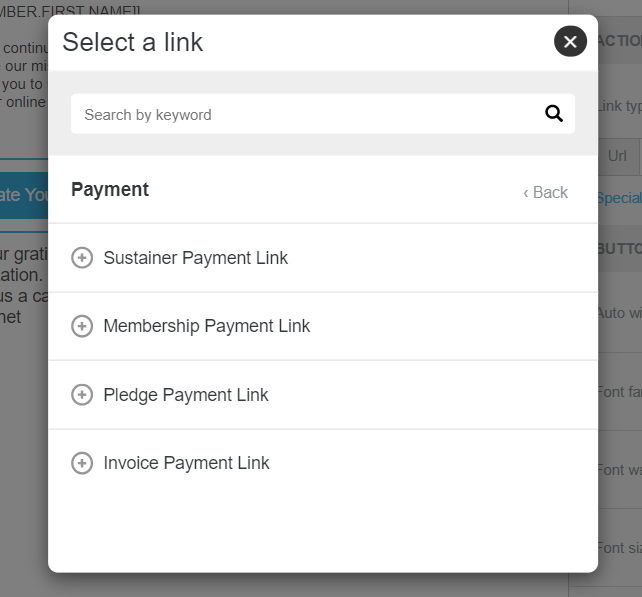This image is a close-up screenshot of a pop-up box displayed on a website overlaid with an opaque dark grey layer, obscuring the background content. The pop-up box is square with rounded corners, featuring the title "Select a Link" in the top left corner. In the top right corner, there is a grey circle containing an "X" icon for closing the pop-up.

Directly below the title, a grey bar hosts a white search bar with the placeholder text "Search by keyword" and a magnifying glass icon on the far right for initiating the search.

The main content of the pop-up appears in a structured, table-like layout with each section separated by thin grey lines. The heading at the top of this layout reads "Payment" in bold text on the left, and "Back" with a left-pointing arrow on the far right. 

Below the heading, the first line includes a circle with a plus sign followed by the text "Sustain a Payment Link." The subsequent lines follow the same format, each starting with a circle and a plus sign and followed by:
- "Membership Payment Link"
- "Pledge Payment Link"
- "Invoice Payment Link"

Each entry is neatly separated by thin grey lines to maintain the organized appearance of the table.